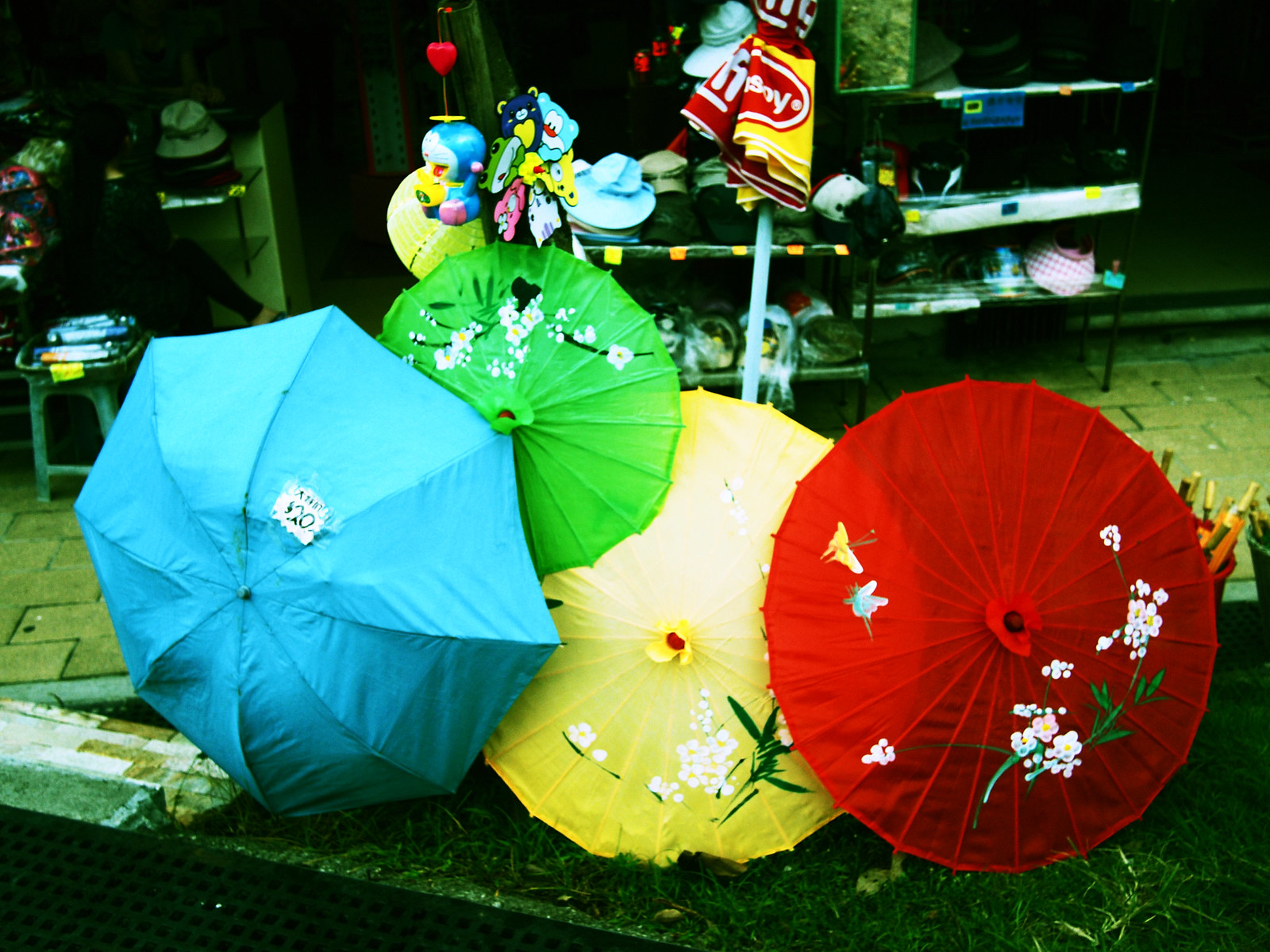This horizontal rectangular photograph appears to be taken outside, possibly in front of a store or inside a mall as indicated by the background. The scene is dominated by a display of open umbrellas laid out on a grassy, triangular planter in the foreground. There are four umbrellas in various colors from left to right: a plain bright blue one with a white price tag reading "$20" in black text, a smaller green umbrella adorned with floral designs, a yellow umbrella also decorated with flowers and a sun-like motif at its center, and a red umbrella featuring floral patterns as well.

Behind the umbrellas, the background consists of gray brick tiles or pavers forming a walkway. Further back, there are black shelving units filled with a miscellany of merchandise including hats, apparel, toys, folded fabrics, and possibly wooden animal cutouts. On the right side of the image, multiple tubs or buckets hold closed umbrellas, adding to the bustling display of goods. There also seems to be a shadow outline of a woman with a ponytail wearing a dark blouse and black leggings, possibly sitting at a counter near the retail area. The crowded and colorful arrangement of items alongside the neatly aligned umbrellas gives the image a vibrant, market-like atmosphere.